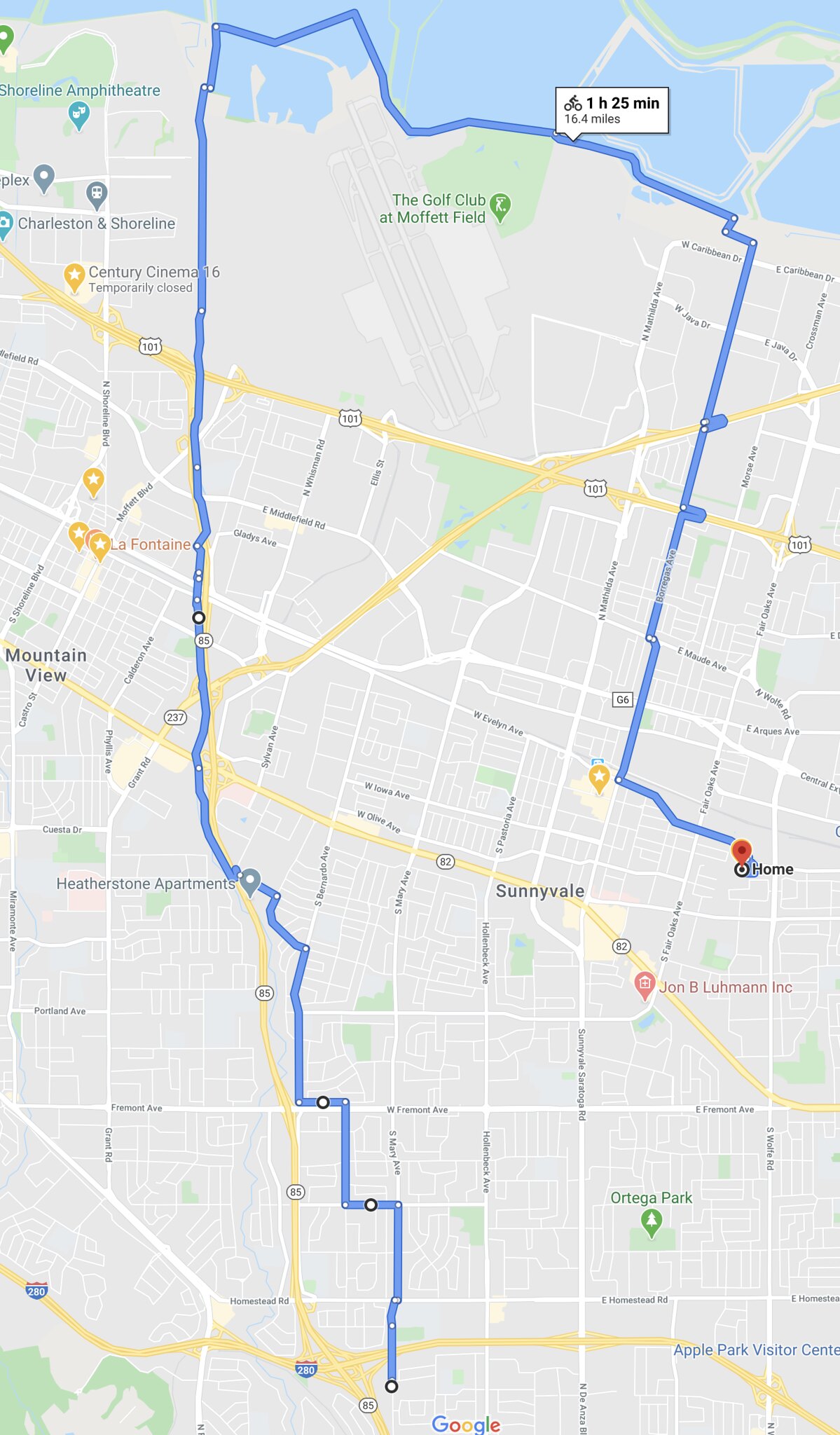The map displayed highlights a detailed cycling route through the Sunnyvale area. The route begins at the bottom of the map, heading northward until it reaches the top boundary. It then curves eastward, following the coastline, before circling back southward to the starting point. A small informational square at the top of the map indicates that the bike route covers 16.4 miles and is estimated to take one hour and 25 minutes. The square includes an icon of a cyclist, emphasizing that it is a bike route.

Key landmarks along the route are marked, including major interstates and highways such as Interstate 280, Highway 85, Highway 82, Highway 237, and Highway 101. The journey primarily follows Highway 85, continuing up to the coastline, where the path extends across the water to the right side of the map. The route then proceeds south, intersecting Highway 101, before reaching its endpoint near John B. Lumen Incorporated and a street name indicating "home."

Other notable locations highlighted on the map include Ortega Park at the bottom right, Sunnyvale city center prominently marked, Mountain View on the far left, Charleston Shoreline, and Moffett Field Golf Club. Hedgestown Apartments are also visible on the left side of the map, alongside various street names, adding further detail to the depicted area.